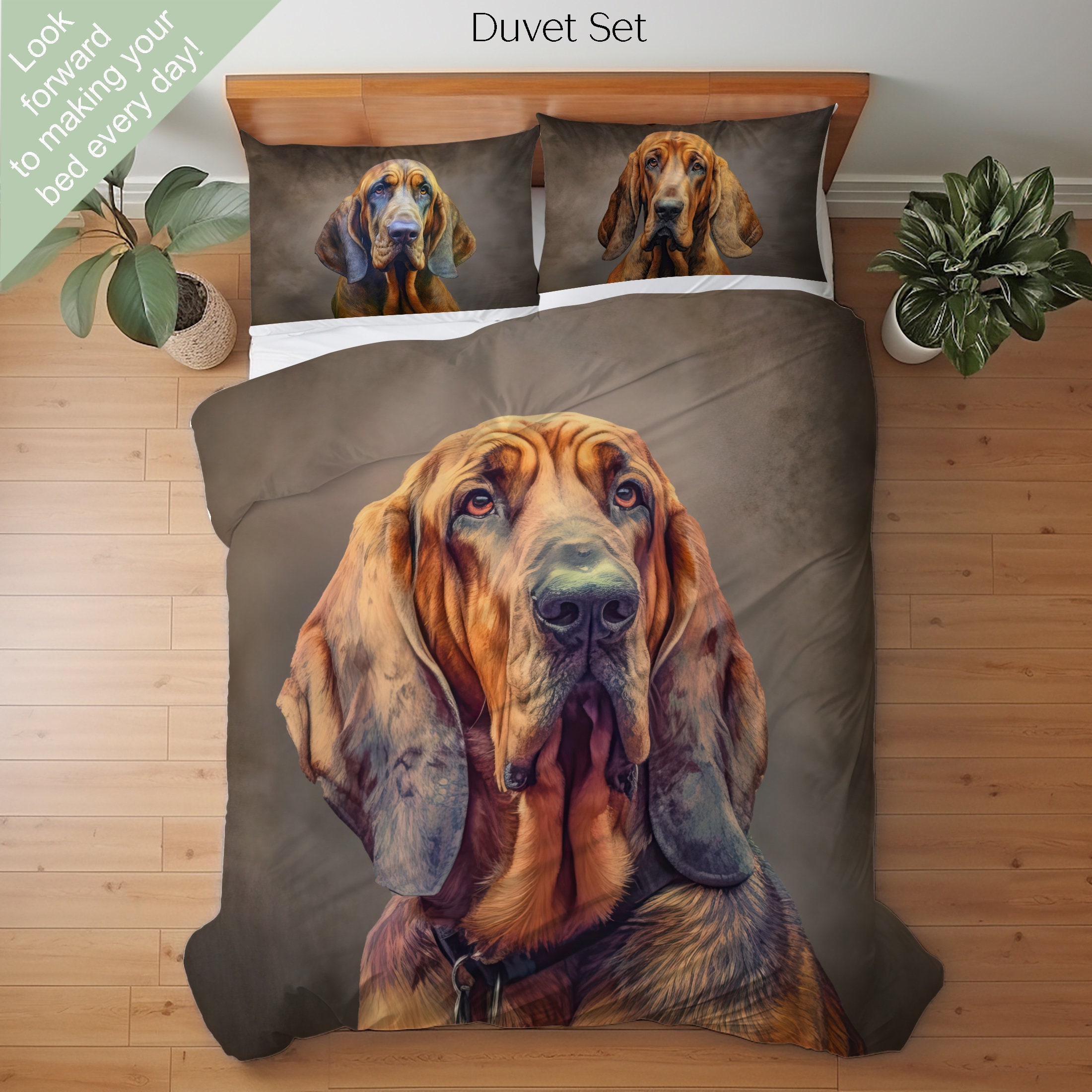This image features an advertisement for a duvet set adorned with photorealistic dog art. The scene is viewed from above, as if from the ceiling, showcasing a bed with a wooden headboard on a pine wood floor against a white wall. Each side of the bed is flanked by a potted plant, both different in type. The duvet cover prominently displays a large, photorealistic painting of a basset hound, characterized by its long ears, brown fur with black highlights, wrinkly sad face, and black nose. Complementing this, the left pillow features a similar image of the basset hound, while the right pillow displays another brown basset hound with no black ear highlights, suggesting it is a different dog. Above, in the upper left corner, a green triangle contains the text, "Look forward to making your bed every day," encouraging viewers to enjoy the playful design. The rooms' sheets are white, adding a crisp contrast to the bold, detailed imagery of the dogs on the duvet set.